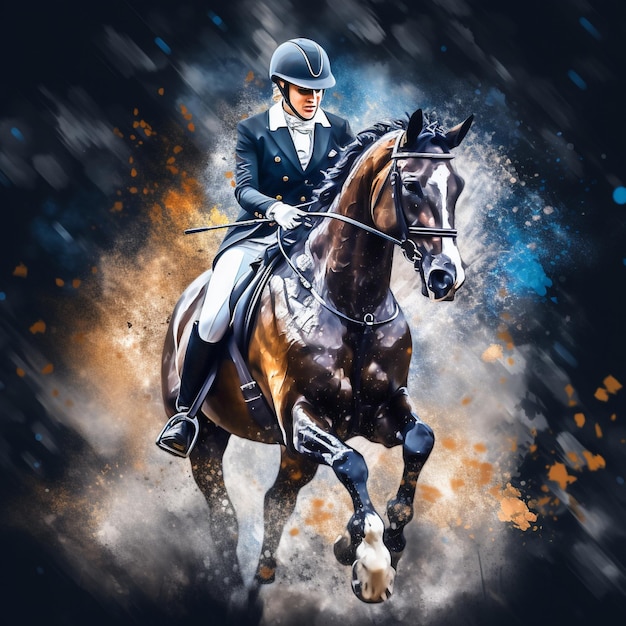The image is a digitally created, vividly detailed painting of a woman jockey riding a brown racehorse with a white stripe along its nose. The jockey, a white woman with blonde hair, is dressed in formal equestrian attire including a blue and white double-breasted suit, white riding pants, black boots secured in the boot holders, and a riding helmet. She holds a whip and the bridle, guiding the horse in mid-gallop, moving slightly toward the right and directly towards the viewer. The background features a dynamic blend of colors—white, blue, grey, orange, tan, and black—creating a blurred, paint-splattered effect that implies motion and speed. The scene around the horse suggests dust kicked up from its powerful run, enhancing the sense of dramatic urgency and elegance in the composition. This image captures the essence of competitive horse racing, possibly symbolizing a significant achievement or honor for the jockey.